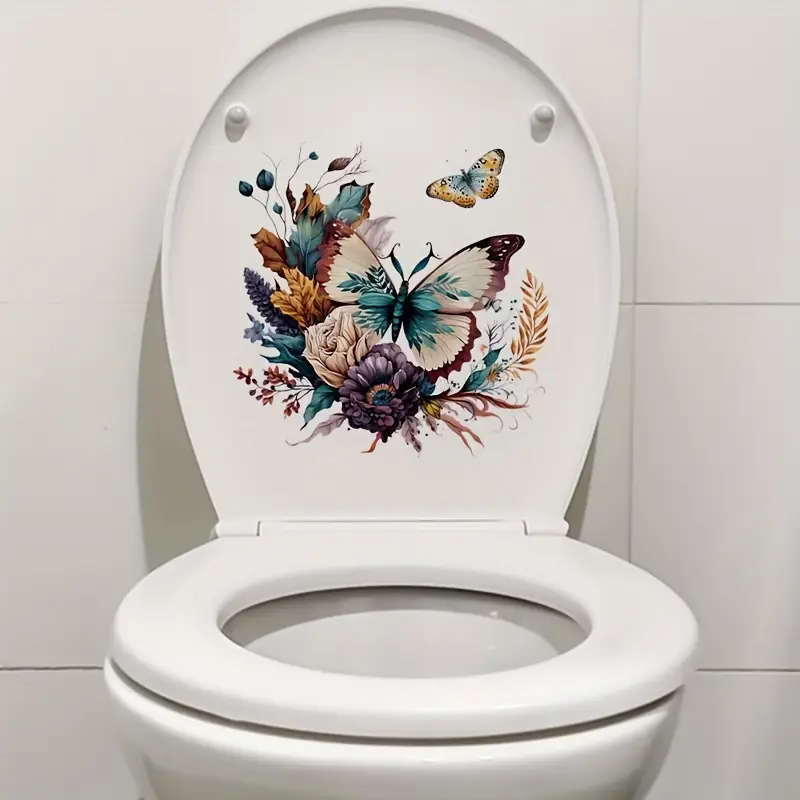This is a detailed photograph of a white toilet with the seat down and the lid up, showcasing an intricate painting on the inside of the lid. The background consists of white tiled walls divided into square sections, enhancing the simplicity and cleanliness of the scene. The standout feature is the beautifully painted illustration on the toilet lid. Dominating the center is a sizable butterfly with white wings edged in maroon and brown tones, and its body is a striking greenish-blue. This butterfly is surrounded by a cluster of flowers and foliage—specifically, a purple flower, a white flower positioned above it, and beige, tan, and brown leaves on either side. Additionally, there is a smaller butterfly in the upper right corner, seemingly in flight, with delicate light blue and yellow shading. Combined, these elements create a vivid and elegant floral design that brings an artistic touch to an otherwise ordinary bathroom fixture.